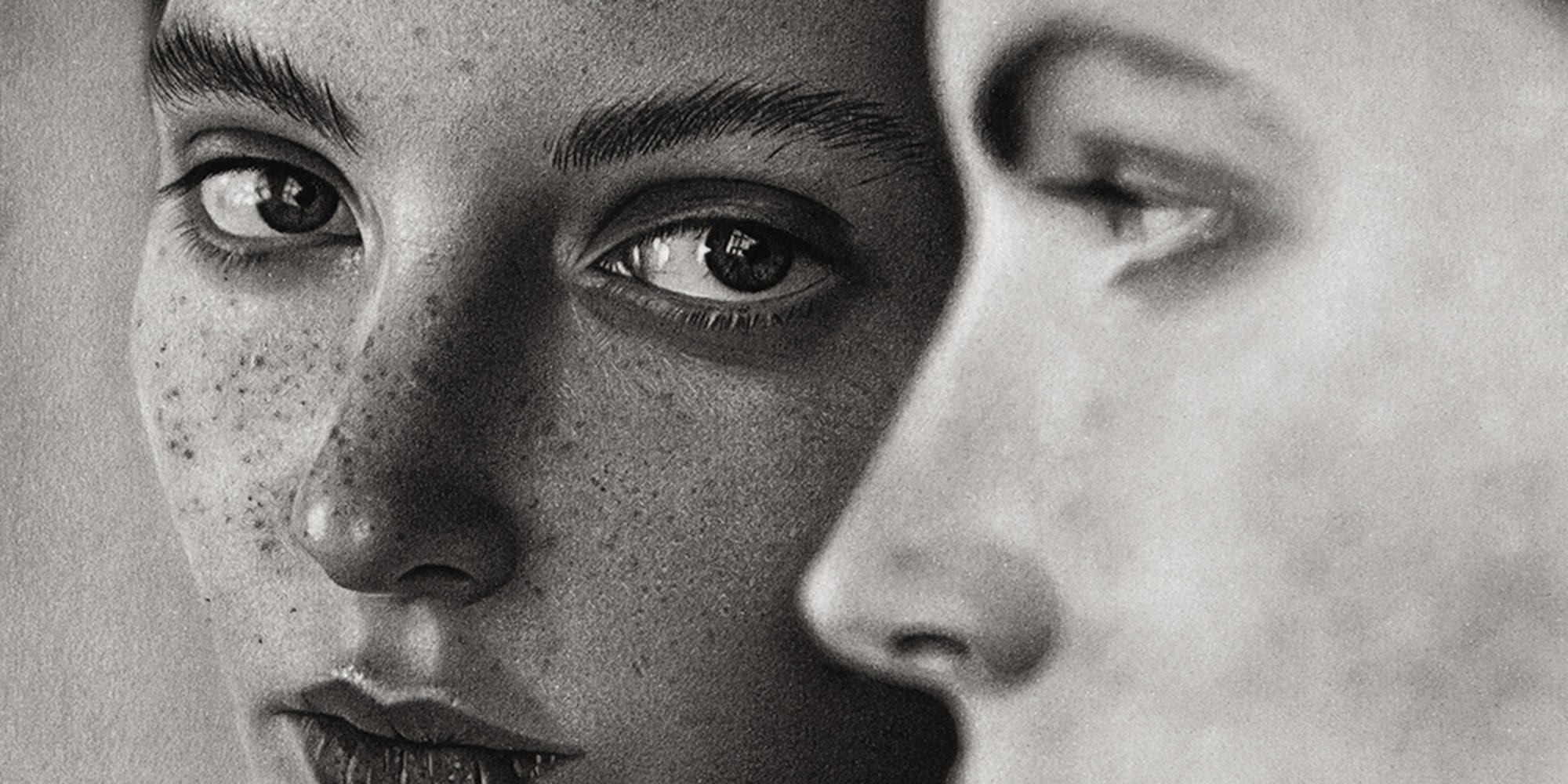The image is a black-and-white (or more accurately, gray-and-white) photograph featuring two women. On the left-hand side, a middle-aged woman with a freckled face, large eyebrows, and pronounced eyelashes stares directly into the camera. She has a darker skin tone compared to the other woman and wears dark-colored lipstick. The detail of the photograph allows her freckles and facial pores to be clearly visible. On the right-hand side, there is another woman with a paler complexion, gazing off to the left, showcasing her profile with an average-sized nose. Her face is slightly more in the foreground, partially obscuring the woman on the left. Both women appear calm and concentrated, contributing to a serene and contemplative mood in the photo.